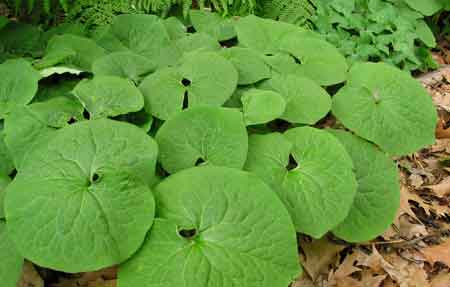The image captures a verdant scene dominated by large, round green leaves reminiscent of lily pads, though they are not in water but rather growing from the ground, supported by stems. The focus is on these prominent leaves, which take up most of the photo, creating a lush display of greenery. Surrounding these central leaves are additional smaller green leaves and possibly fern-like plants contributing to the scene's rich vegetation. In contrast, the bottom right of the photo features a cluster of dry, brown fallen leaves, adding a touch of autumnal decay to the vibrant green of the primary plants. The overall feeling conveyed is one of abundant, diverse foliage with intricate textures and a blend of living greenery and decayed leaves, indicating an outdoor setting.